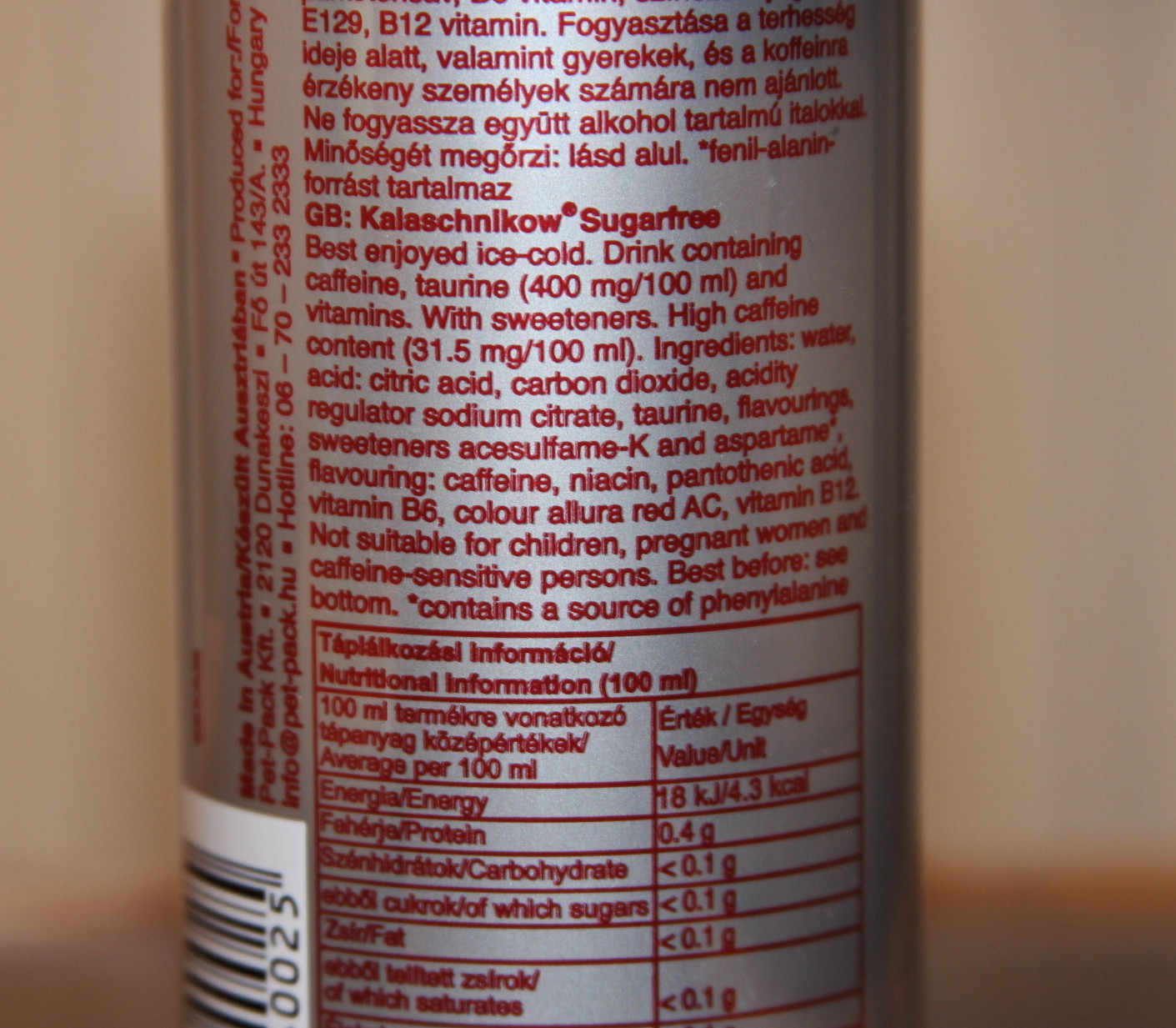The image depicts a close-up, color photograph of a partially visible beverage can. The focus is on the silver metallic surface of the can, which occupies about three-quarters of the image's width and the entire height. The can's background is a gradient of beige-brown, lighter at the top and transitioning to a darker, shadowy area at the bottom, possibly indicating a floor area with orange and gray hues. The can itself is predominantly silver with text written in maroon.

The text on the can provides detailed information about the beverage, starting with some text in an unidentified language followed by "G.B. Kalashnikov sugar-free. Best enjoyed ice-cold." The drink contains caffeine, taurine (400 mg/100 ml), and vitamins, along with sweeteners. The small maroon lettering also lists ingredients such as water, citric acid, carbon dioxide, acidity regulator (sodium citrate), taurine, flavoring, sweeteners (including acesulfame K and aspartame), and vitamin B12. It is noted that the drink has a high caffeine content of 31.5 mg/100 ml and is not suitable for children, pregnant women, or caffeine-sensitive individuals. Additionally, there is a warning about it containing phenylalanine. Part of the can includes a formal nutritional information table and a vertical text area that is difficult to read. On the bottom left edge, a partially visible barcode with the digits "0025" is present.